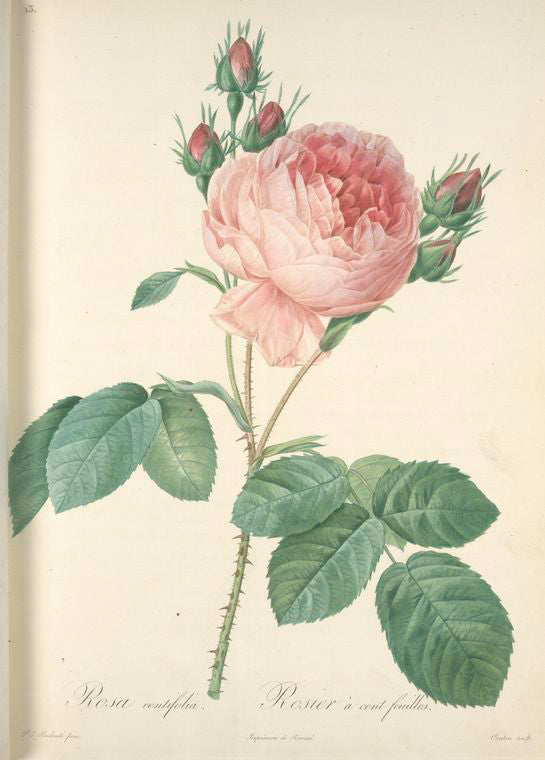This off-white, cream-colored vintage advertisement-like painting, rendered by artist Pierre-Joseph Redouté, features a meticulously detailed pink Rosa Centifolia, also known as Rosier D. Province. The central focus of the artwork is a large, elegant pink rose with five smaller buds sprouting from the sides—three on the left and two on the right. The rose’s thorny stem supports lush, green leaves with serrated edges that enhance the botanical accuracy of the image. Some shading on the sides adds depth to the petals and leaves, giving the piece a lifelike quality. At the bottom of the painting, elegant black script identifies the flower as "Rosa Centifolia," underscoring its exquisite beauty and historical significance.